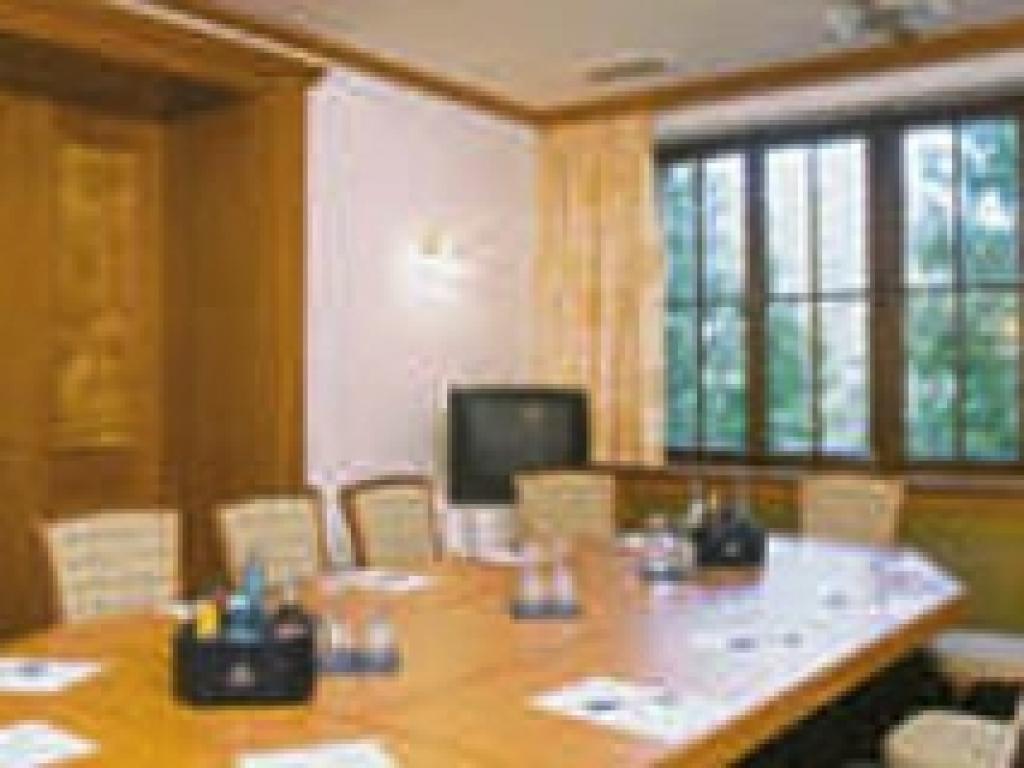The image depicts a partially blurry, highly pixelated scene, making it difficult to determine if it's a photograph or an illustration. The focus is a large dining room or kitchen area, with a light-colored wooden dining table dominating the foreground. The table is surrounded by seven chairs, each with tan-colored fabric backs. Scattered around the table are items that appear to be placemats or menus, along with black plastic holders containing condiments like sauces, and possibly salt and pepper shakers or sugar containers, suggesting a restaurant or hotel setting rather than a private home.

In the upper right portion of the image, a large window with multiple rectangular panes and a brown windowsill is visible. Green trees can be glimpsed outside, indicating a pleasant view. Light brown or off-white curtains hang on the left side of the window. The white ceiling features brown decorative trim along the edges.

To the left side of the image is a closed, brown wooden door suggesting an entry or exit point. Behind the table, set against the white wall, stands an older model television from the 1980s or 1990s, placed on a small table or stand. The overall scene hints at a spacious room, cleanly decorated, possibly for communal gatherings.